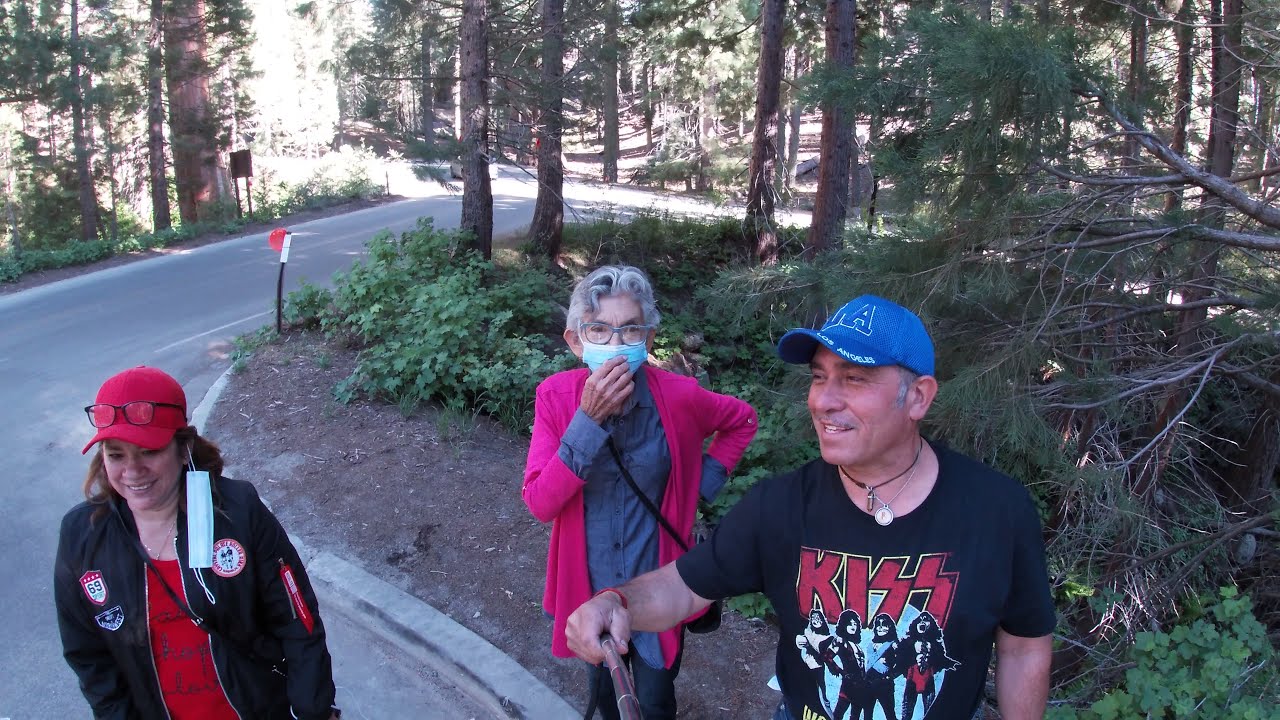The image is a vivid color photograph, captured in landscape orientation, featuring a selfie of three people standing on a paved trail in a wooded area. The man on the right, who is holding the selfie stick in his right hand, is wearing a blue Los Angeles Dodgers baseball cap and a black KISS band t-shirt. He has two necklaces around his neck and is looking away to the side, smiling. In the center of the photo is an older woman with gray hair and glasses, wearing a pink sweater over a gray long-sleeve shirt and a crossbody bag. She has a face mask on and appears to be adjusting it as she looks up at the camera. To the far left stands another woman, smiling, in a black zip-up jacket over a red shirt, with a red baseball cap that has her glasses perched on top. She has a dangling face mask from her left ear. The background features a curved paved path with a tree island and more forested areas, portraying a serene and realistic outdoor setting.